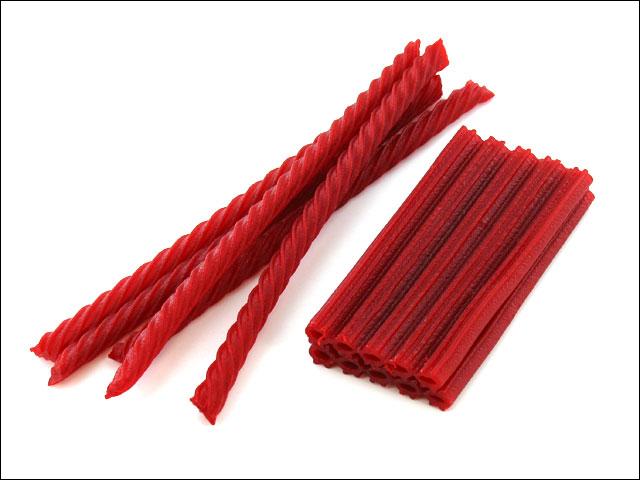In this image, set against a completely white background with a thin black border, there are two groups of red Twizzlers (a type of red licorice candy). On the left side, there are five Twizzlers that appear loosely lying on top of each other, with two of them slightly overlapping at a shallow angle, almost intersecting the right side group. To the right, there are ten Twizzlers neatly stacked together in a log-like arrangement. These right-side Twizzlers remain connected, forming a cohesive bundle. The image contains no text or other objects, highlighting the contrasting arrangement of the Twizzlers: the more chaotic left side and the orderly right side.